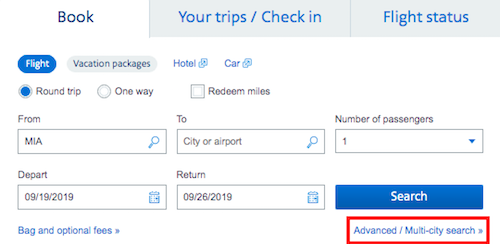Screenshot Description: 

The screenshot depicts a flight booking page on an undisclosed website, viewed on a PC. The interface is minimalistic, predominantly white, with most text elements in blue, apart from a single red instance. 

- **Top Navigation**:
  - The top edge is designed like file folder tabs. The active tab is labeled 'Book' in blue, while two other tabs, 'Your Trips/Check-In' and 'Flight Status,' are indicated with pale blue backgrounds and darker blue text.

- **Main Booking Section**:
  - Below the top navigation, the first line contains a blue-highlighted button labeled 'Flight' in white text. Adjacent buttons with pale blue backgrounds offer additional options: 'Vacation Packages,' 'Hotel,' and 'Car'.
  - The next line features trip options: 'Round Trip' (selected), 'One Way,' and a checkbox for 'Redeem Miles'.
  
- **Flight Details**:
  - Following lines include input fields:
    - 'From' with placeholder 'MIA' and a search feature.
    - 'To' for the destination city or airport.
    - Number of passengers, currently set to one.
  - Departure and return dates are filled in as '09/19/2019' and '09/26/2019' respectively.

- **Search and Additional Options**:
  - A blue button labeled 'Search' in white text is prominently displayed.
  - Below this button, in red text with blue print, is a link for 'Advanced/Multi-City Search'.
  - On the lower left corner of the same line, small blue text reads 'Bag and Optional Fees'.

This organized structure directs users effortlessly through the steps required to book a flight, from selecting trip types to entering specific flight details.